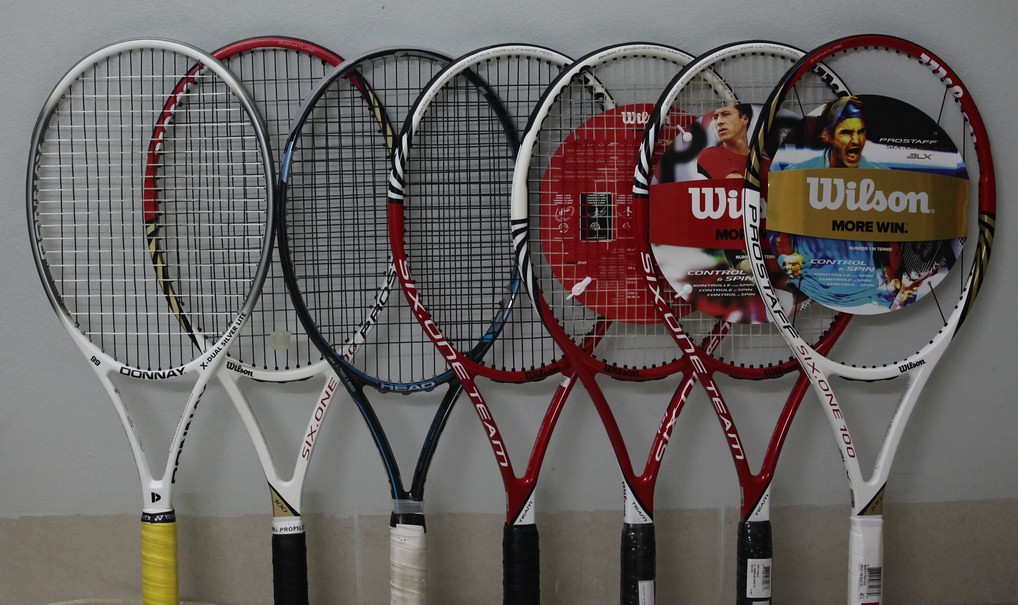The image showcases seven tennis rackets leaning against a white and brown wall. The rackets feature an array of colors and branding. Three primarily white rackets include one with a yellow handle, one with a black handle, and one with a white handle and "Pro Staff 6-100" written on it, which still has the Wilson packaging displaying the name "Moore Wynn." There's a blue racket with a white handle that also states "Head." Among the three red tennis rackets with black handles, all marked "6-1 Team," two retain their Wilson wrappers. Overall, the brands and writing on the rackets include "Donnell," "6-1 Pro," "Head," and the red ones specifically indicate "Wilson Control Spin" and feature different player images, one of which is Roger Federer. All the rackets are overlapping each other, creating a visually engaging display.